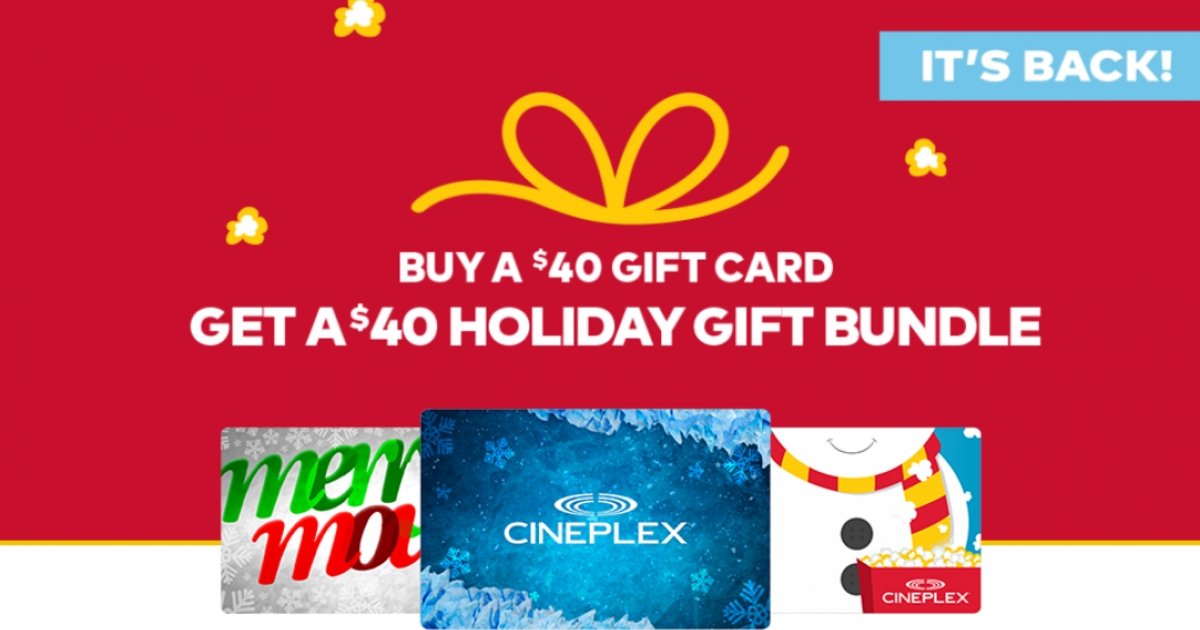This is a promotional screenshot from an unknown web page with a festive, red-themed background decorated with illustrations of popcorn kernels—two on the left and one on the right. In the top right corner, there is a prominent blue banner with white text declaring, "It's Back!" At the center of the image, a yellow drawing of a gift bow grabs attention. Directly below the bow, bold white text reads, "Buy a $40 gift card. Get a $40 holiday gift bundle."

Towards the bottom of the image are three distinct gift card images, each showcasing unique holiday designs. The leftmost card, partially obscured, features a silver background adorned with a snowflake pattern and festive green and red writing. The central gift card displays a chilly blue background with white ice and snowflake motifs, with "Cineplex" written in striking white letters at the center. The third card, on the right and also partially covered, depicts a smiling snowman donning a red and yellow striped scarf. Adjacent to this is a vibrant red Cineplex popcorn box, with pieces of popcorn cascading into it from above.

Overall, the image blends fun holiday elements with promotional content, focusing on gift cards and the bundled offer without depicting any people.